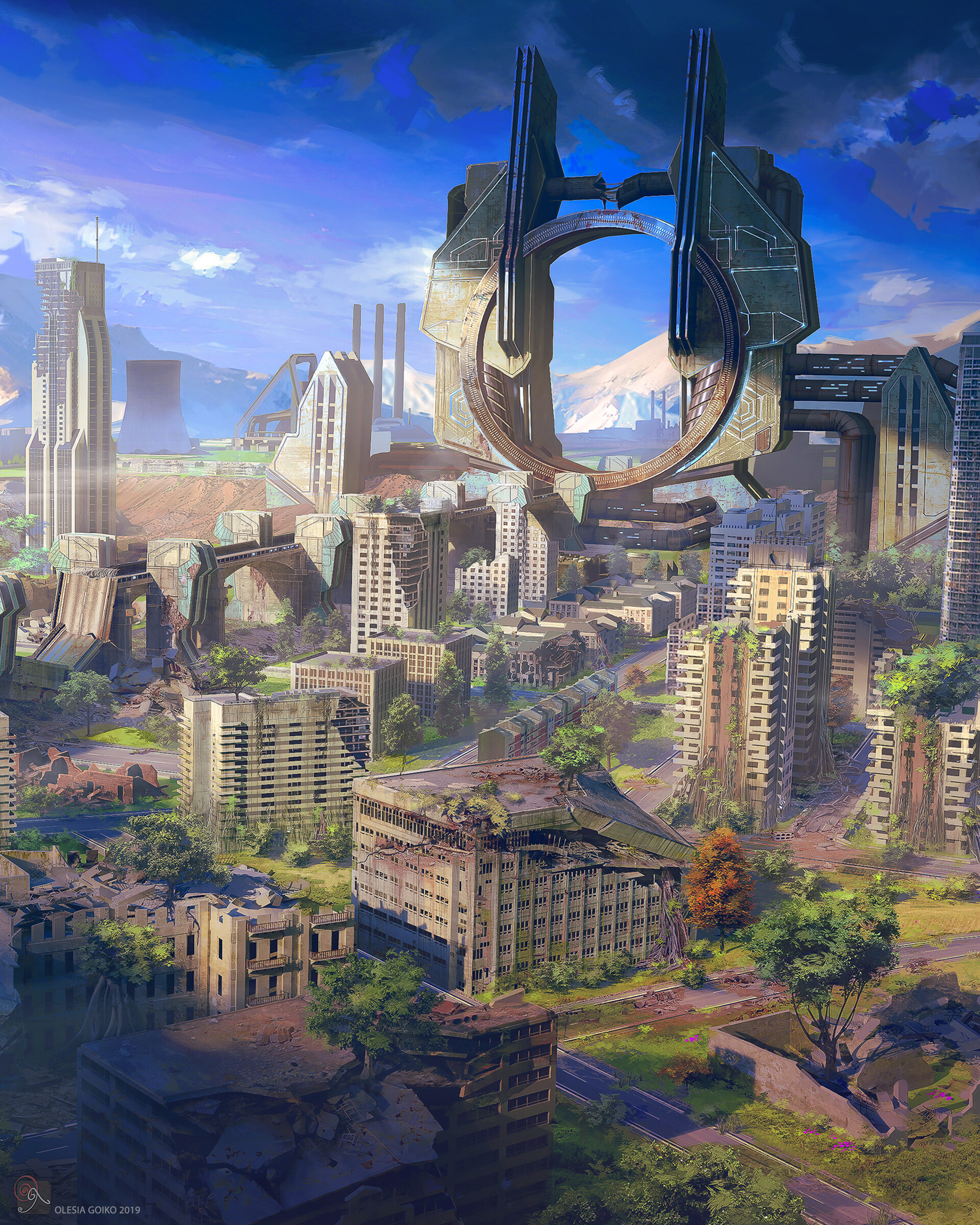The image showcases a detailed, cartoonish painting of a futuristic yet dystopian cityscape, appearing to be abandoned and overgrown with foliage. The city is filled with tall, gray high-rise buildings, some of which are visibly collapsing and covered in greenery, indicating significant decay and neglect. Trees and grass have overrun the structures, seeping through the cracks and crevices. In the foreground, there's a peculiar floating spaceship-like structure, characterized by a large circle with two prongs pointing skyward, possibly part of an alien invasion, featuring pipes connecting to the city's infrastructure. A nuclear power plant can be seen in the background, beneath a blue sky dotted with white clouds. The perspective of the image is at an angle, almost resembling a bird's eye view, capturing the full extent of the deserted, post-apocalyptic environment. The overall scene conveys a striking contrast between technological advancement and natural reclamation, providing a haunting glimpse into a possible future where nature reclaims a once-bustling metropolis.